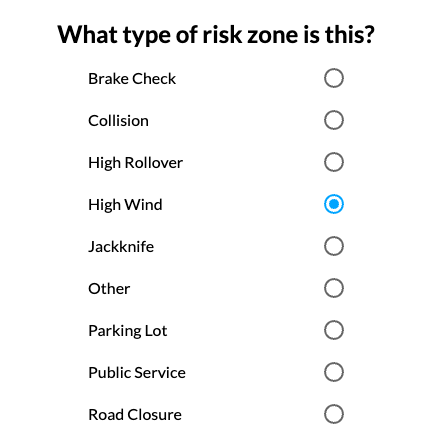This image features a simplistic design with a white background. There are no photographs, drawings, or additional graphics present. The text is rendered entirely in black, providing a stark contrast against the plain backdrop. The layout appears in a rectangular format, notably taller than it is wide.

At the top of the image, bold text reads, "What type of risk zone is this?". Below this heading, there are nine options listed vertically, each followed by an unfilled circle except for one which has a blue-filled center. Here are the options in detail with their corresponding circles:

1. **Break check** - Empty circle
2. **Collision** - Empty circle
3. **High rollover** - Empty circle
4. **High wind** - Blue-filled circle
5. **Jackknife** - Empty circle
6. **Other** - Empty circle
7. **Parking lot** - Empty circle
8. **Public service** - Empty circle
9. **Road closure** - Empty circle

The single blue-filled circle next to "High wind" indicates the selected or active risk zone among the given options.